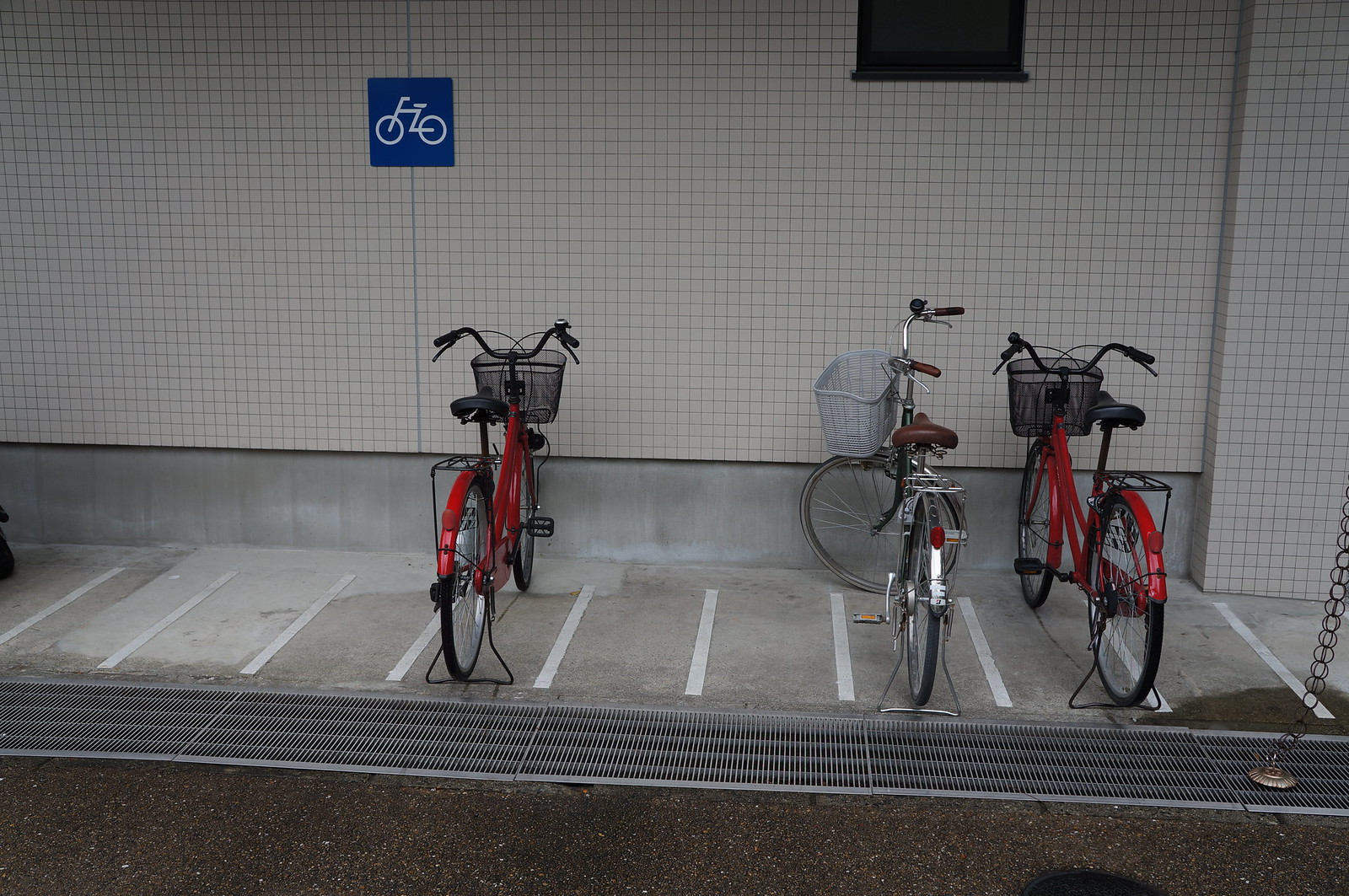The image showcases a neatly organized bicycle parking area against a backdrop of a white tile wall composed of small squares. Three classic roadster-style bikes are parked in designated stalls, which are demarcated by narrow stripes slightly wider than a typical sidewalk. The bicycles are lined up facing the wall, revealing their back tires. Two of the bikes are red with black seats and feature handle brakes and front baskets, while the bike in the middle has a silver frame, a brown seat, and a white basket. A blue sign bearing a white bicycle symbol is visible on the left side of the image, indicating the bicycle parking area. Below this sign, a rain chain is noted, suggesting efficient water drainage into a metal grate installed behind the bikes. The scene is slightly wet, likely due to recent rain. In the upper right corner, the wall features a small black window. The overall setting suggests a location possibly in Asia or Japan, given the distinct design elements.